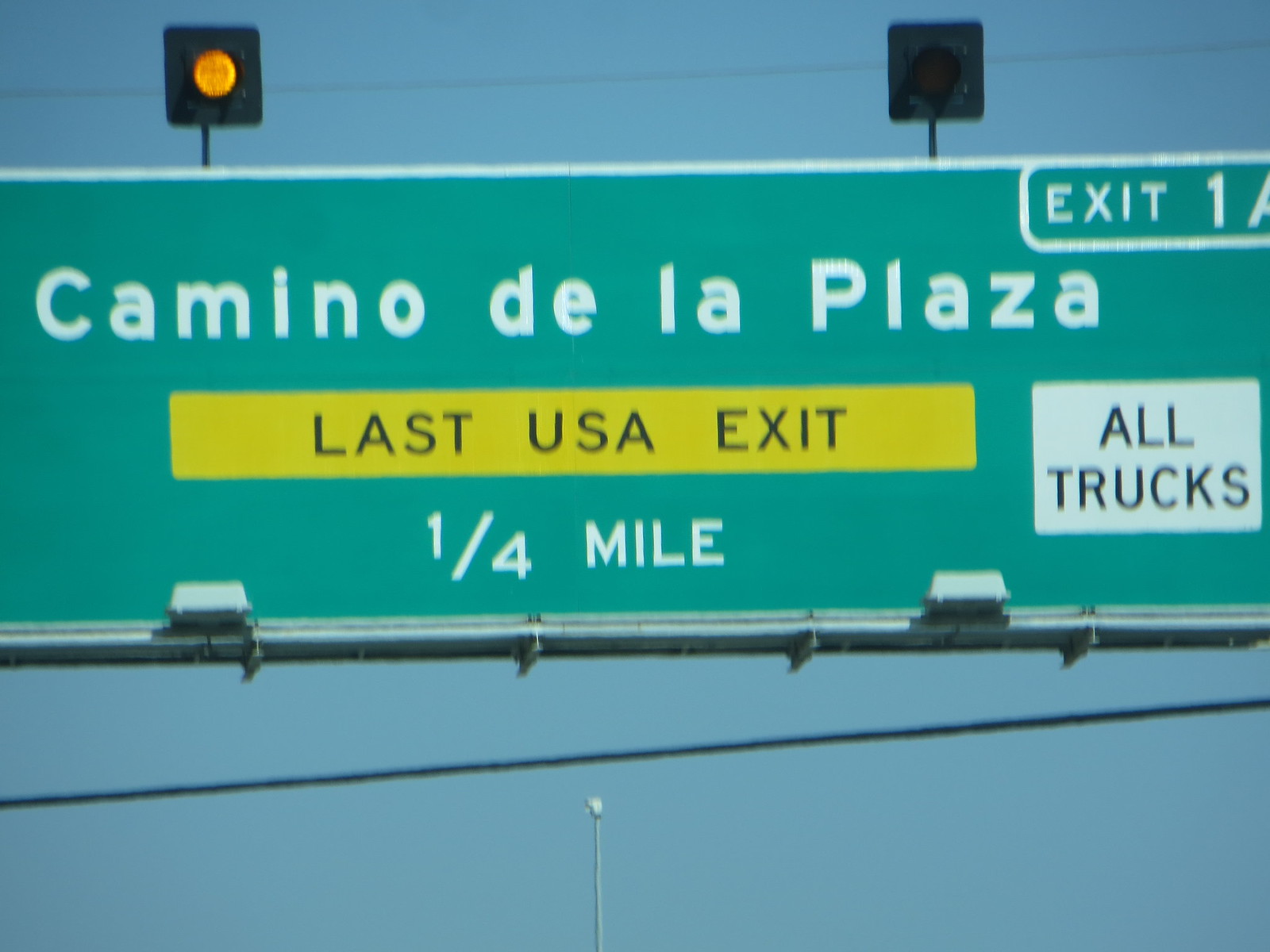The image features a close-up view of a highway sign against a clear blue sky. The sign has a green background, prominently displaying the text "Camino de la Plaza" in large, white letters. Centered within the green portion of the sign is a yellow box with the black text "LAST USA EXIT." Below this, the distance "1/4 MILE" is noted in smaller white text. On the left side of the sign, the designation "EXIT 1A" is inscribed, though the letter 'A' is partially cut off in the middle.

Additionally, there's a white box with the text "ALL TRUCKS" in black letters located near the bottom of the sign. Two yellow blinking lights are attached to the top of the sign; one light is illuminated while the other is off. The image shows a streetlamp seemingly emerging from beneath the sign and several wires: one positioned atop the sign and another descending diagonally from right to left at approximately a 30-degree angle. The focus on the detailed elements of the highway sign emphasizes its importance as an alert for the last exit before the border.